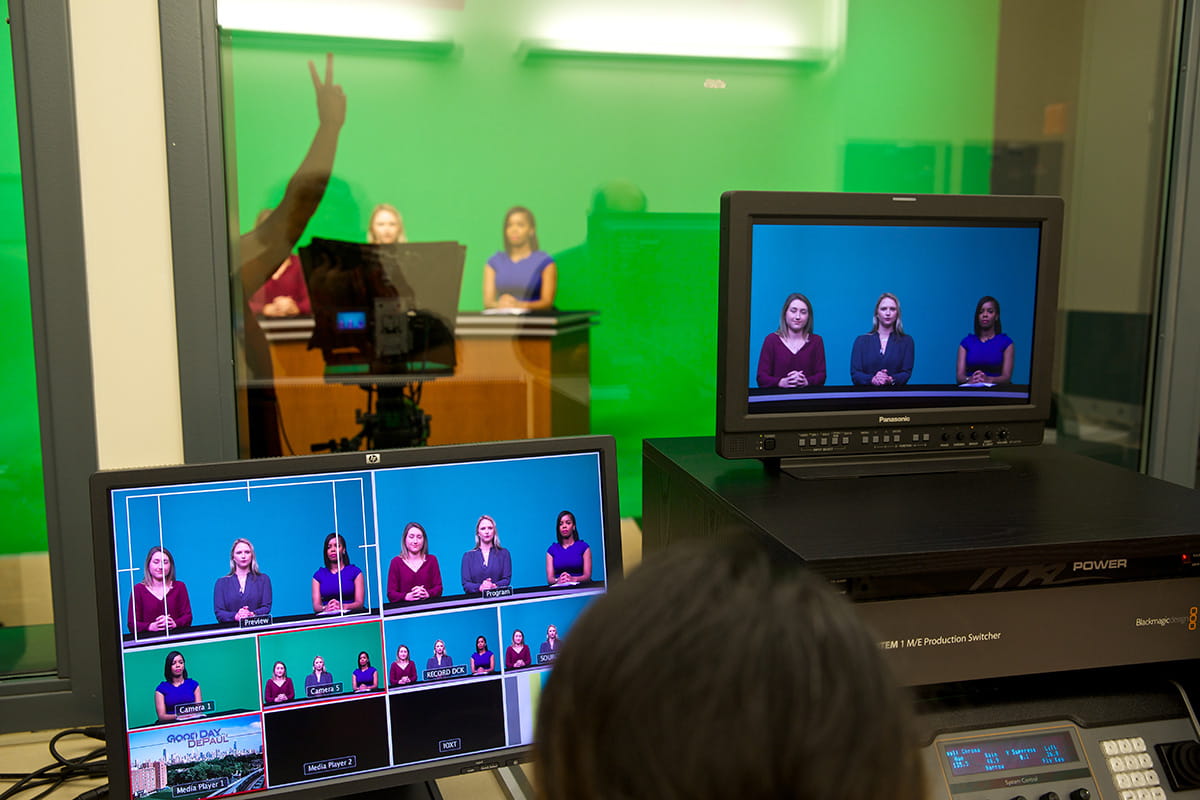The image captures an indoor scene of a TV studio’s production booth, focusing on the behind-the-scenes activities of a local news broadcast. In the foreground, there is the back of a person’s head, who is seated and looking at two computer monitors. The left monitor displays multiple camera views, each showcasing three women dressed in formal attire, seated at a table with their hands folded – sometimes highlighted individually and sometimes collectively, all in front of a blue screen. The right monitor sits atop complex electrical equipment and shows similar images alongside labeled camera views.

Further back, through a glass window, a person near a camera is holding up a peace sign with two fingers extended. Behind them is a large green screen where the same three women seen on the monitors are actually seated at a desk, partially obscured by the technical setup. Various colors, including bright green, burgundy, blue, dark purple, black, white, beige, and tan, are visible throughout the scene, reflecting the lively atmosphere of the studio. The backdrop features a cityscape with "Good Day DePaul" displayed prominently, indicating this is likely a set for a local news show.